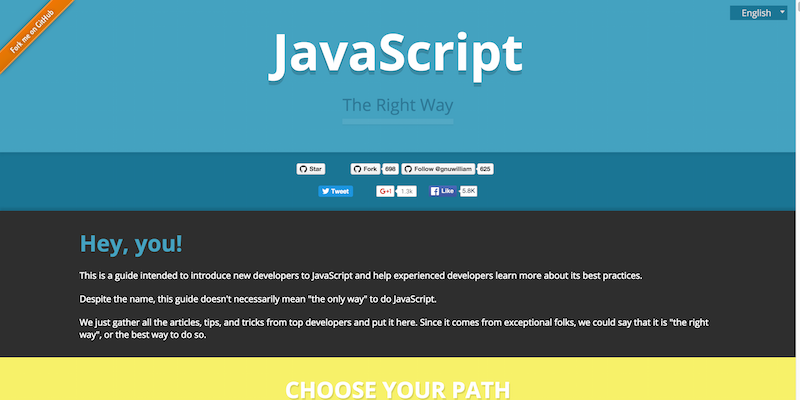Here's a detailed, cleaned-up caption for the described image:

---

The webpage features a JavaScript-themed layout with a visually distinctive blue background dominating the top half. In the upper left corner, an orange diagonal banner with white text reading "Fork Me on GridHub" extends toward the top right corner. Centrally positioned, bold white text displays the word "JavaScript," with smaller, darker blue text underneath stating "The Right Way." 

In the upper right corner, there is a darker blue rectangle with white text reading "English" next to a drop-down menu button. Below the blue background section, there's a horizontal darker blue rectangle in the center containing interactive elements. 

In the middle of this rectangle are several black-text rectangles. The first rectangle reads "Star," followed by another that says "Fork," and then the phrases "GenuWilliam" and "625." Further down, a blue rectangle contains white text saying "Tweet" next to a white rectangle with red text that reads "G+1." This is followed by another white rectangle with black text that states "1.3K," and finally, a Facebook "Like" button.

Continuing below, the background turns black, and on the left, blue text announces "Hey You." Below this, white text explains that the guide aims to introduce new developers to JavaScript and assist experienced developers in refining their practices. The text emphasizes that while the guide is thorough, it is not the only way to approach JavaScript. The assembled articles, tips, and tricks come from top developers, suggesting that it represents the right or best way.

At the bottom, a yellow rectangular band stretches across the width of the page, featuring white text that reads "Choose Your Path."

---